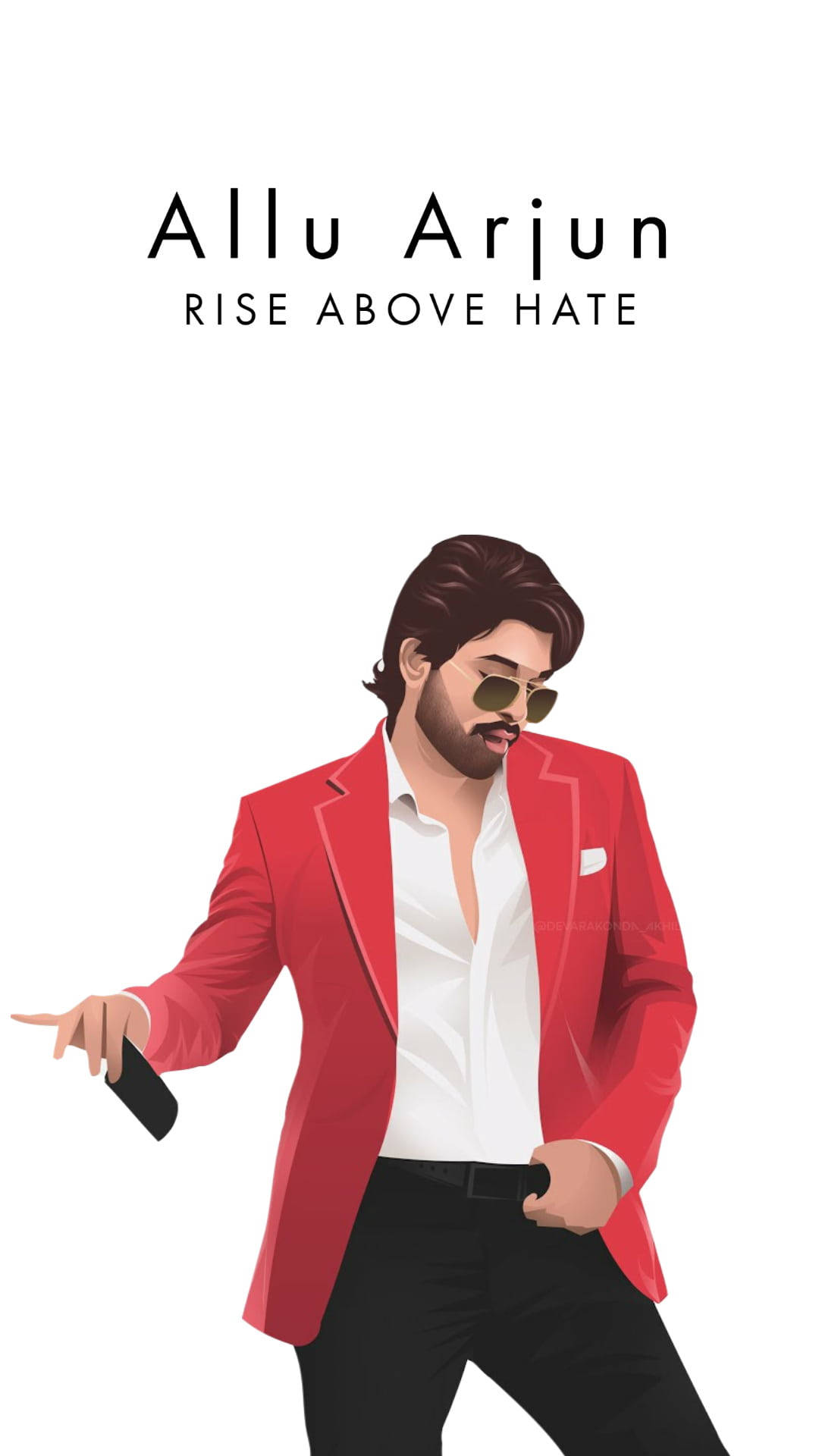This digital illustration appears to be an advertisement, possibly for a music album or an upcoming concert, featuring the entertainer Allu Arjun. The artwork depicts a young, light brown-skinned male with dark brown, well-groomed hair, neatly brushed back, and a trimmed beard and mustache. His head is inclined towards the bottom right corner, and he sports sunglasses that enhance his stylish look. Allu Arjun is dressed in sleek black pants, a partially unbuttoned shiny white shirt, and a striking red dinner jacket. His left hand is hooked into his pants line, propping open his blazer, while his right hand holds a black rectangular object, likely a credit card, in a distinctive pose. The text at the top of the advertisement reads "Allu Arjun" in bold black letters, followed by "Rise Above Hate," against a white background. This carefully detailed vector illustration captures Allu Arjun’s suave and provocative stance, amplifying his celebrity persona.